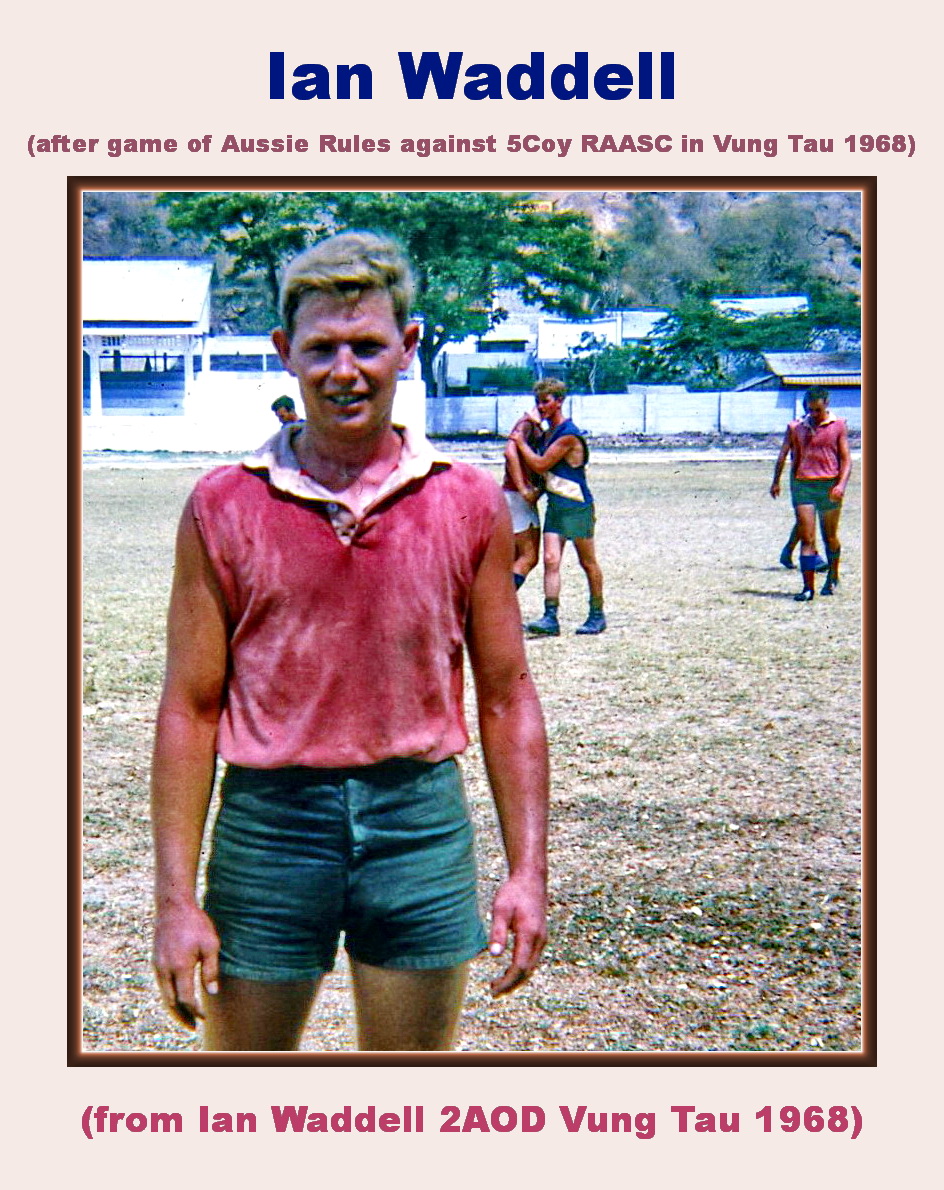The photograph is an aged but colorful image encased in a picture-frame-like border with a gray background and a thin brown edge. At the top of the border, the blue text reads "Ian Waddell," while pink text beneath states "After Game of Aussie Rules Against Five Koi R.A.A.S.C. in Vung Tau, 1968." The bottom of the border features another line in pinkish text: "From Ian Waddell to A.O.D., Vung Tau, 1968."

In the center of the image, several men are playing a sport in a flat green field. Prominently featured in the foreground is a man wearing a sleeveless t-shirt with a collar and short blue jean shorts. The players wear red cutoff-sleeved shirts, hinting at a team uniform. The scene is set in an outdoor complex with a white wall and lush green trees in the background, resembling an older stadium or sports facility. The photograph appears to capture a moment post-game, reflecting the era of 1968 with its vibrant yet nostalgic tones.